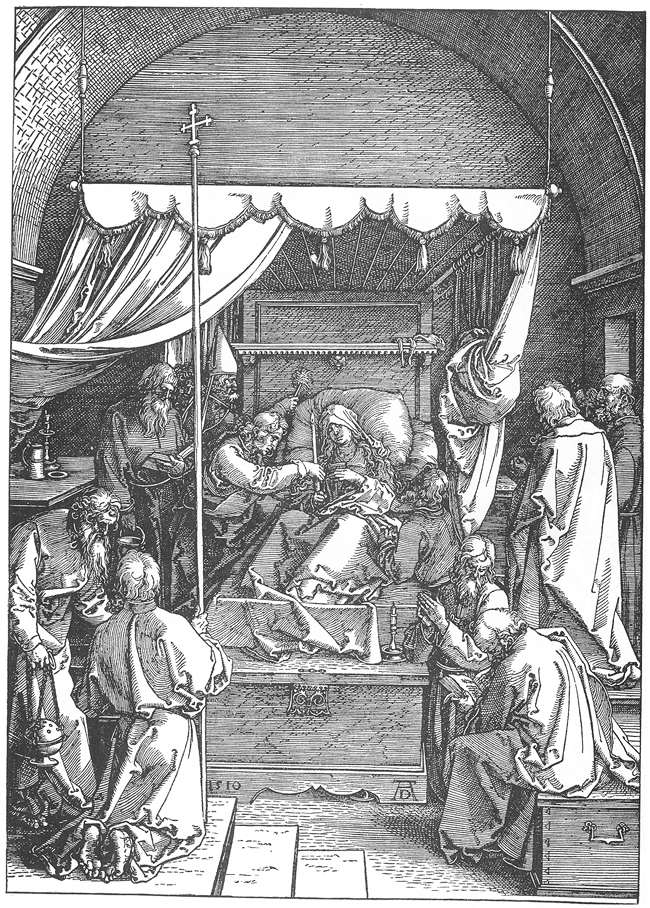This black and white sketch, likely rendered in pencil or pen, depicts a historic scene set within an old building, possibly from the 1600s or 1700s. The arched ceiling is meticulously detailed with hatched lines, creating a sense of depth and grandeur. At the center of the composition is a woman reclining on a bed with white drapings and elaborate pillows, suggesting she might be ill. She holds a candle in her right hand and rests against the cushions, her head adorned with a headband. 

Surrounding her are several men, most dressed in long religious robes with some donning bishop hats, indicating a religious context. One man to her left leans over, perhaps in a gesture of comfort, while another reads from a book, possibly a Bible. In the foreground, a man kneels in prayer while another speaks to him. Several of the men are carrying lanterns with chains and holding sticks topped with crosses. The grandeur and solemnity of the scene are heightened by the small details like the chest on the floor and stair steps leading up to the bed, emphasizing the significance of the moment portrayed in the drawing.